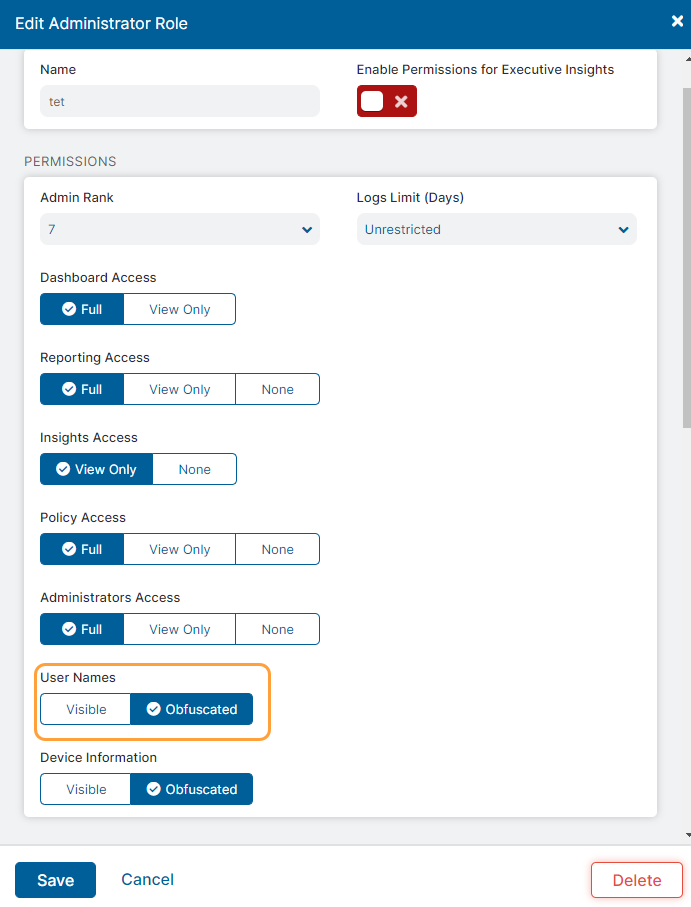The image displays a webpage featuring settings for editing an administrator role. At the top, there's a blue banner with the title "Edit Administrator Role." Below it, the field "Name" is labeled "Name Tent Name" with a grey entry box for text input against a white background.

To the right, there's an option to "Enable Permission for Executive Insights," marked by a red box with a check mark and an 'X’. 

Further down are various permissions settings, each in boxes on a white background:

- **Admin Rank:** Set at 7.
- **Log Limits:** In days, unrestricted.
- **Dashboard Access:** Options for view-only or none, view-only is currently selected.
- **Reporting Access:** Options for view-only or none, with view-only selected.
- **Insights Access:** Options for view-only or none, with view-only selected.
- **Policy Access:** Options for view-only or none.
- **Administrators Access:** Options for view-only or none.

There are also options to make usernames and device information either visible or obfuscated.

At the bottom of the webpage, there are three buttons labeled "Save" (in blue), "Cancel," and "Delete."